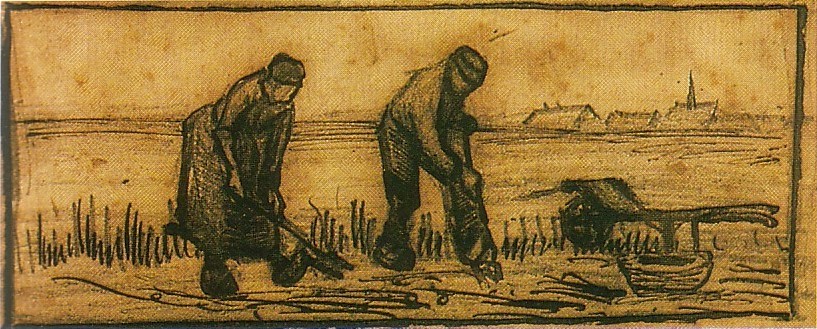A wide, rough pencil or charcoal sketch on a light sepia background depicts a scene of farm labor, likely in the form of tilling the soil. The artwork features minimal detail, with the human figures relegated to shaded silhouettes devoid of facial features. Centered in the composition are a man and a woman; the woman is positioned on the left, while the man is to her immediate right. Both are hunched over, engrossed in their work. The man is dressed in a long-sleeved shirt, long pants, and a short-billed cap, while the woman wears a dress and a hat. Each of them clasps a shovel, angled as if they are in the act of digging. To their right is farm equipment, including a wheelbarrow or cart and a round bucket. The field around them appears freshly tilled, with short grass and shrubs directly behind. In the distant background, a steepled building, likely a church, and two adjacent buildings punctuate the otherwise level and even terrain.